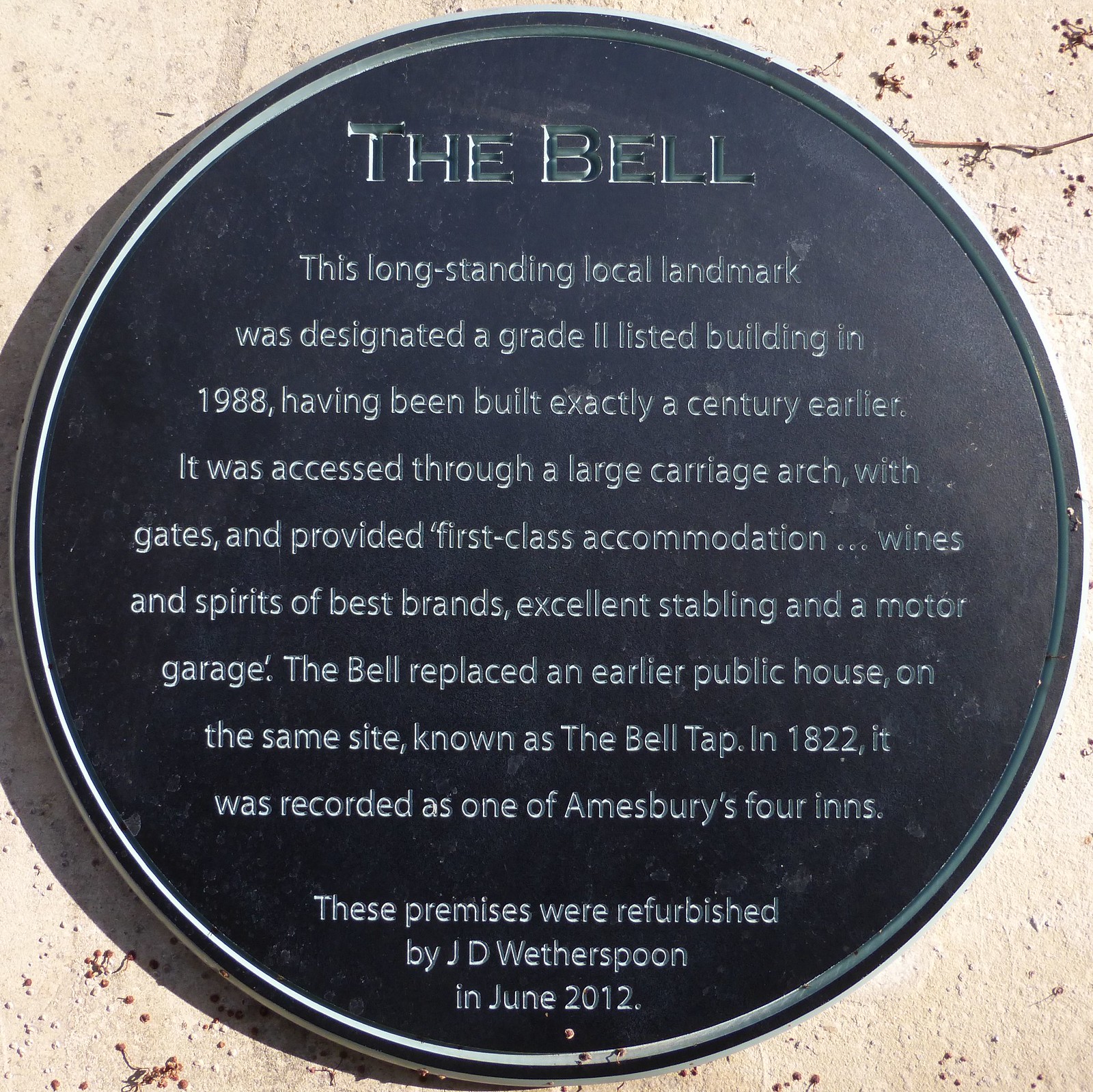The photograph features a round, black plaque with white inscriptions, prominently mounted on a beige stone wall, recessed within the stone. The circular plaque has a dark green line around its outer edge, and it is titled "The Bell" at the top. The detailed text inscribed on the plaque explains that "The Bell," a long-standing local landmark, was designated a Grade II listed building in 1988, having been constructed a century earlier in 1888. Originally accessed through a large carriage arch with gates, the establishment offered first-class accommodation, wines and spirits of the best brands, excellent stabling, and a motor garage. "The Bell" replaced an earlier public house on the same site known as "The Bell Tap." In 1822, it was recorded as one of Amesbury's four inns. The premises underwent refurbishment by J.D. Wetherspoon in June 2012.